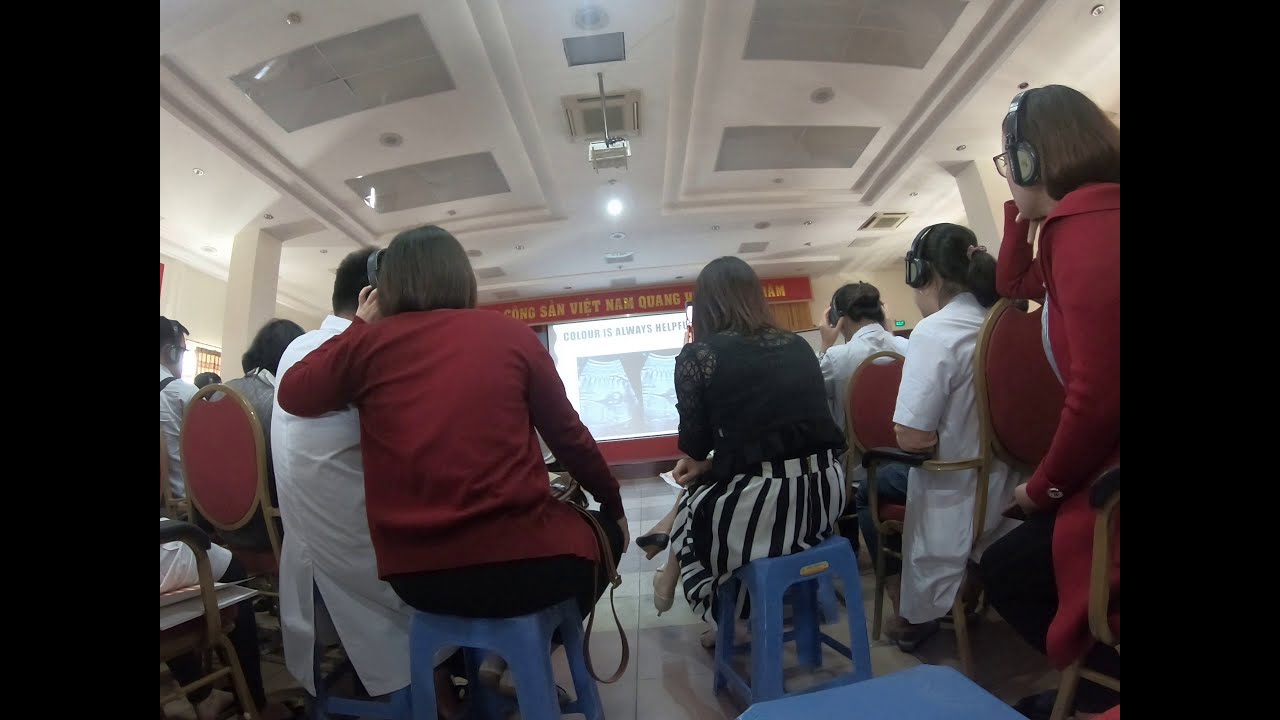The detailed photograph depicts a classroom hall filled with numerous individuals sitting on blue stools and brown seats with red backs and seat surfaces. The image is taken from behind the audience, who are all facing a large screen at the front of the room. Displayed on the screen, likely using a white ceiling-installed projector, is an image that includes partially visible text mentioning "Vietnam." The ceiling, a clean white, features several rectangular skylights and vents. The floor is tiled in white, enhancing the room's bright ambiance.

The attendees, appearing to be engaged in a meeting or presentation, wear headphones and are dressed in variously colored shirts, predominantly white, red, and black. Notably, a woman in a black and white striped skirt is perched on a blue stool, interacting with a nearby man in a white lab coat. Adjacent to her are several other women—one in a red hoodie layered over a white jacket—and a man who seems to be adjusting his headphones. The meticulously detailed room setup and the attendees' attire and positioning suggest a formal, focused environment conducive to concentrated listening and participation.